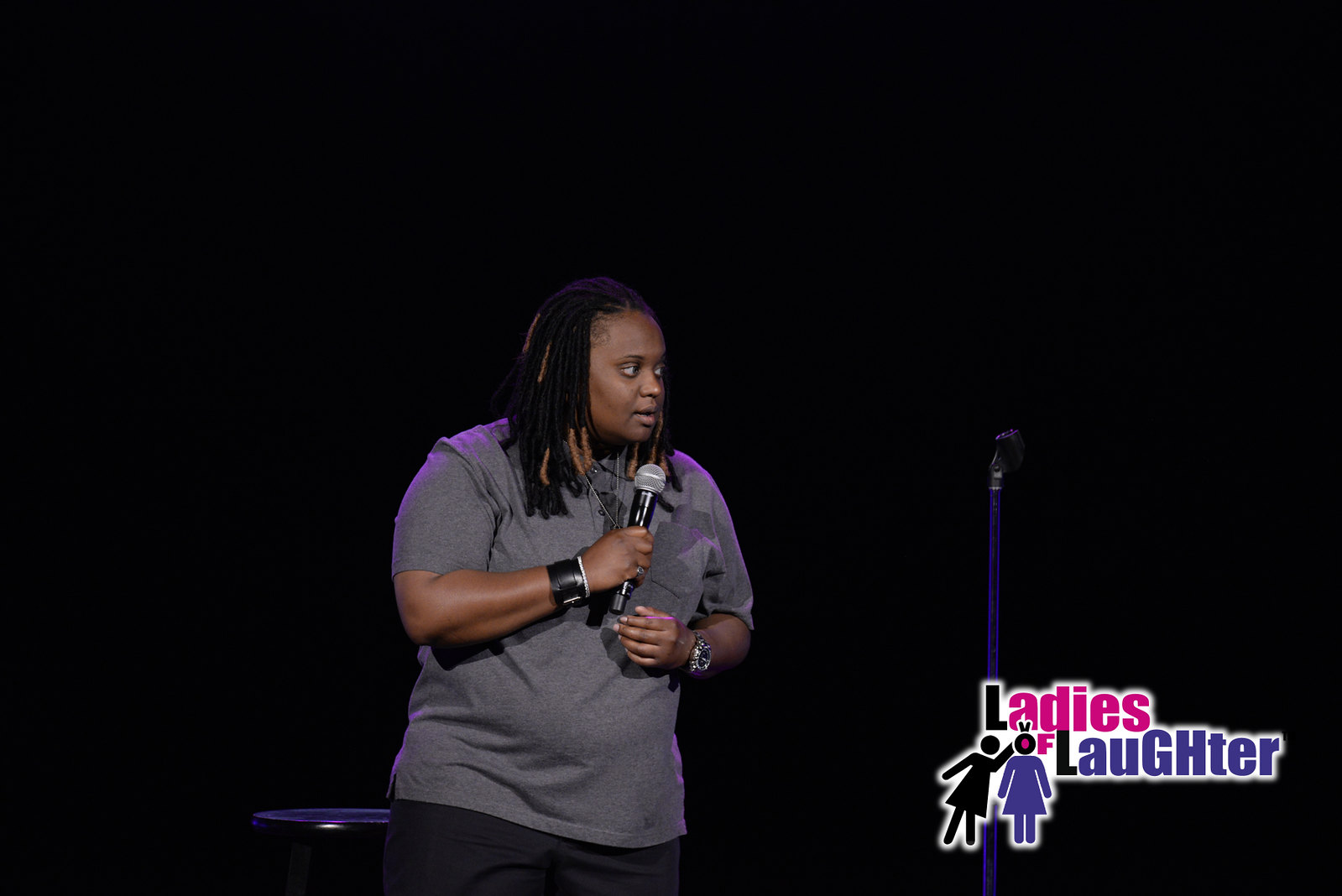A woman stands on a stage with a completely black background. Clad in a short-sleeved gray t-shirt and dark-colored trousers, she holds a microphone in her right hand. Her hair is styled in black plaits, with some brown strands intertwined at the ends. On her left wrist, she wears a watch. To her right, there is a microphone stand, and behind her, partially visible, is a black stool. A subtle purple backlight accents the top and back of her shoulders, creating a slight glow. In the lower right corner of the image, there is a logo featuring silhouettes of two women: one black and the other purple. The text accompanying the logo reads "Ladies of Laughter," with the "O" in "of" represented by the head of the purple silhouette. The logo integrates both black and pink colors for the lettering.